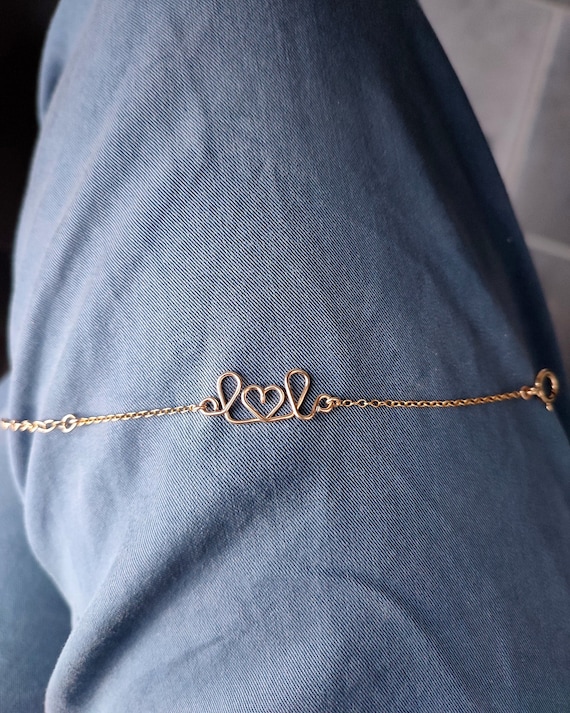The colour photograph captures a close-up view of someone's bent knee clad in slightly wrinkled light blue jeans. Draped across the leg is a golden necklace, with a series of intricate details. The necklace features a chain that runs across the center of the image, adorned in the middle with two loops forming an L shape on either side, and a heart shape connecting the loops resembling the formation "LOL". The clasp and potentially adjustable end suggest it might be a bracelet rather than a full-length necklace. In the blurred background, part of a white wall and a gray door are visible along with a shadow cast on the left side. The upper left corner shows a hint of black, and to the right, the setting appears less illuminated, giving a contrast between shadow and light. There are no other objects or writings present in the picture.